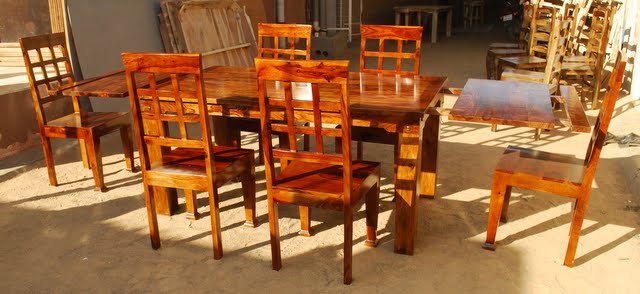This image depicts a family-sized wooden dining table set within an unfinished or partially constructed outdoor area that resembles a storage space or undeveloped room. The table is a dark brown and has a long rectangular shape with two extensions at each end that can be pulled out to make it longer. It is set at a slight angle and bathed in sunlight, casting intricate shadows on the ground beneath. Surrounding the table are six chairs, two on each side and one at each end. The chairs are made from a matching wooden material, featuring open, square-patterned backs. The setting around the table appears cluttered with building materials, suggesting that this space is part of a developing structure, giving an impression of where a dining area would be placed once construction is complete. The ambient sunlight accentuates the glossy finish of the wood, adding to the scene's warm, rustic appeal.